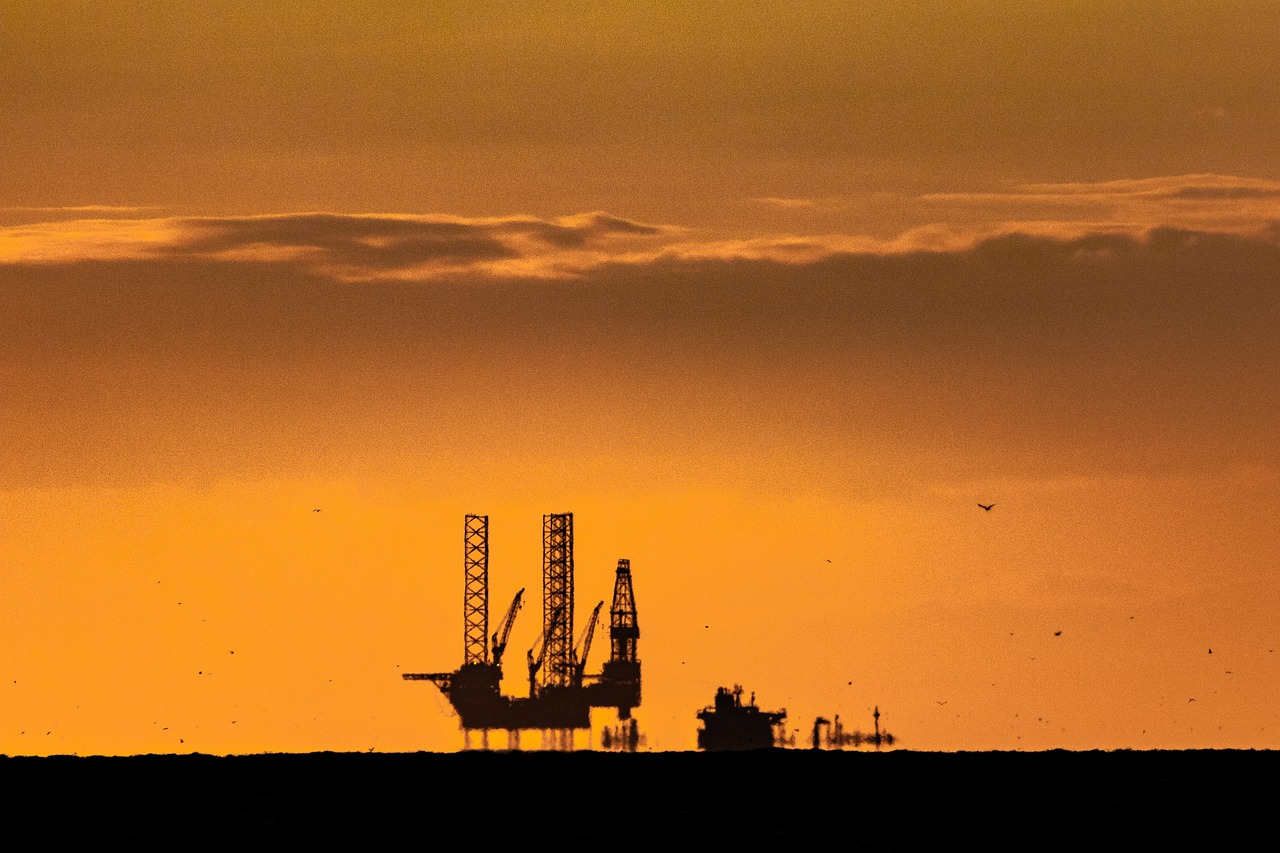The image is a horizontal rectangular photograph capturing a dark, offshore drilling area at sunset. At the very bottom, there's a thin horizontal band that appears black, which is likely water but could also be mistaken for land. Above this, the expansive sky dominates the scene, transitioning from a golden hue at the horizon to a darker, cloud-covered upper portion in shades of brown, gray, and orange. The horizon is adorned with silhouetted structures: primarily an offshore oil platform with three tall towers extending from a base elevated on stilts. To the right of this platform, there's a smaller, less defined structure that might be the front end of a ship. In keeping with the dark, silhouetted theme, the entire scene is subtly detailed with a few birds flying in the distance, adding to the overall serene yet industrial atmosphere of the photograph.